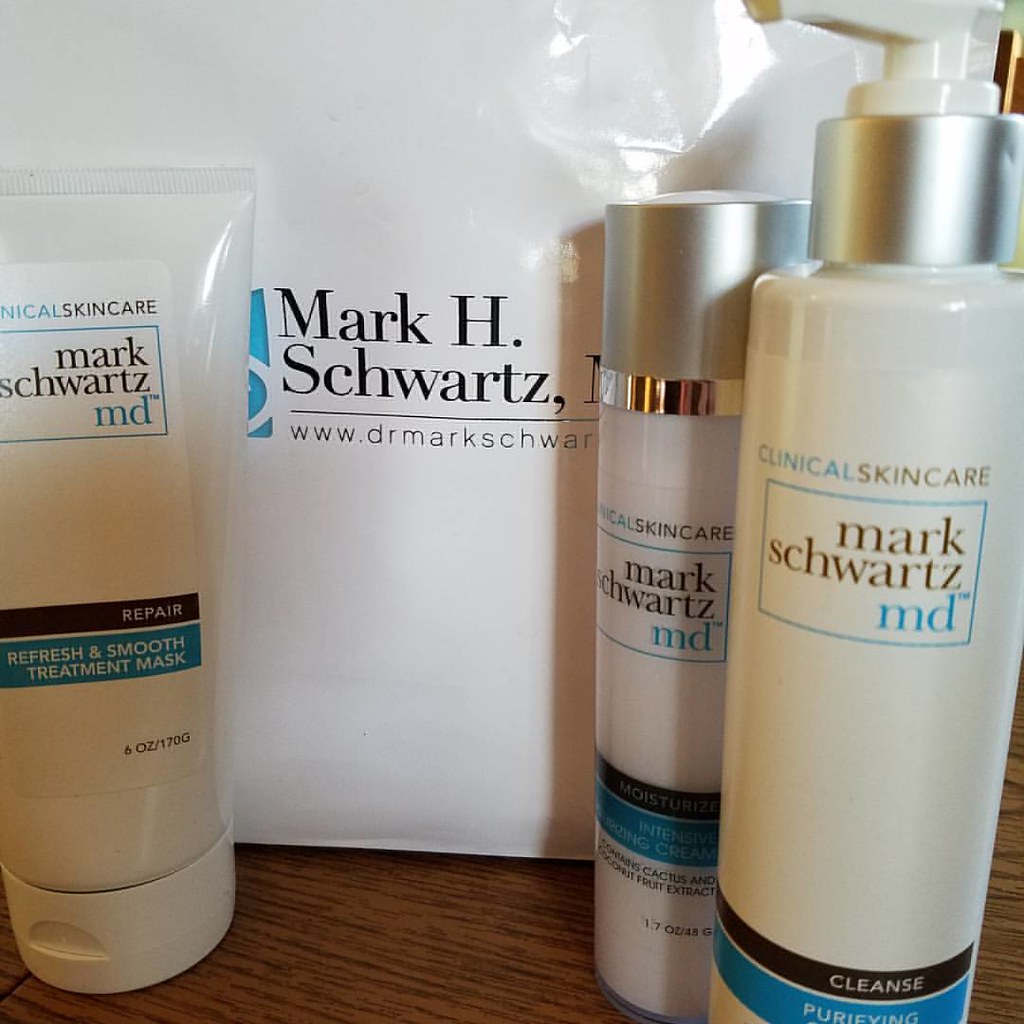The image displays an assortment of clinical skincare products by Mark H. Schwartz, MD, arranged on a brown wooden surface. Dominating the background is a white bag featuring the name "Mark H. Schwartz" along with his website beneath a prominent black line. To the left, there is a partially visible tube adorned with a teal logo, and the text "Clinical Skin Care, Mark Schwartz, MD" near the top. Below this, it continues with "Repair" in a black rectangle followed by "Refresh and Smooth Treatment Mask" in a blue rectangle. Near the center, another tube is positioned with a silver cap, displaying similar branding: "Clinical Skin Care, Mark Schwartz, MD," but its detailed text is somewhat obscured. On the right-hand side, a third product, which appears to be a pump bottle, also showcases the branding "Clinical Skin Care, Mark Schwartz, MD" with "Cleanse and Purifying" inscribed at the bottom. Each product maintains a consistent design, emphasizing the skincare lineup by Mark Schwartz.